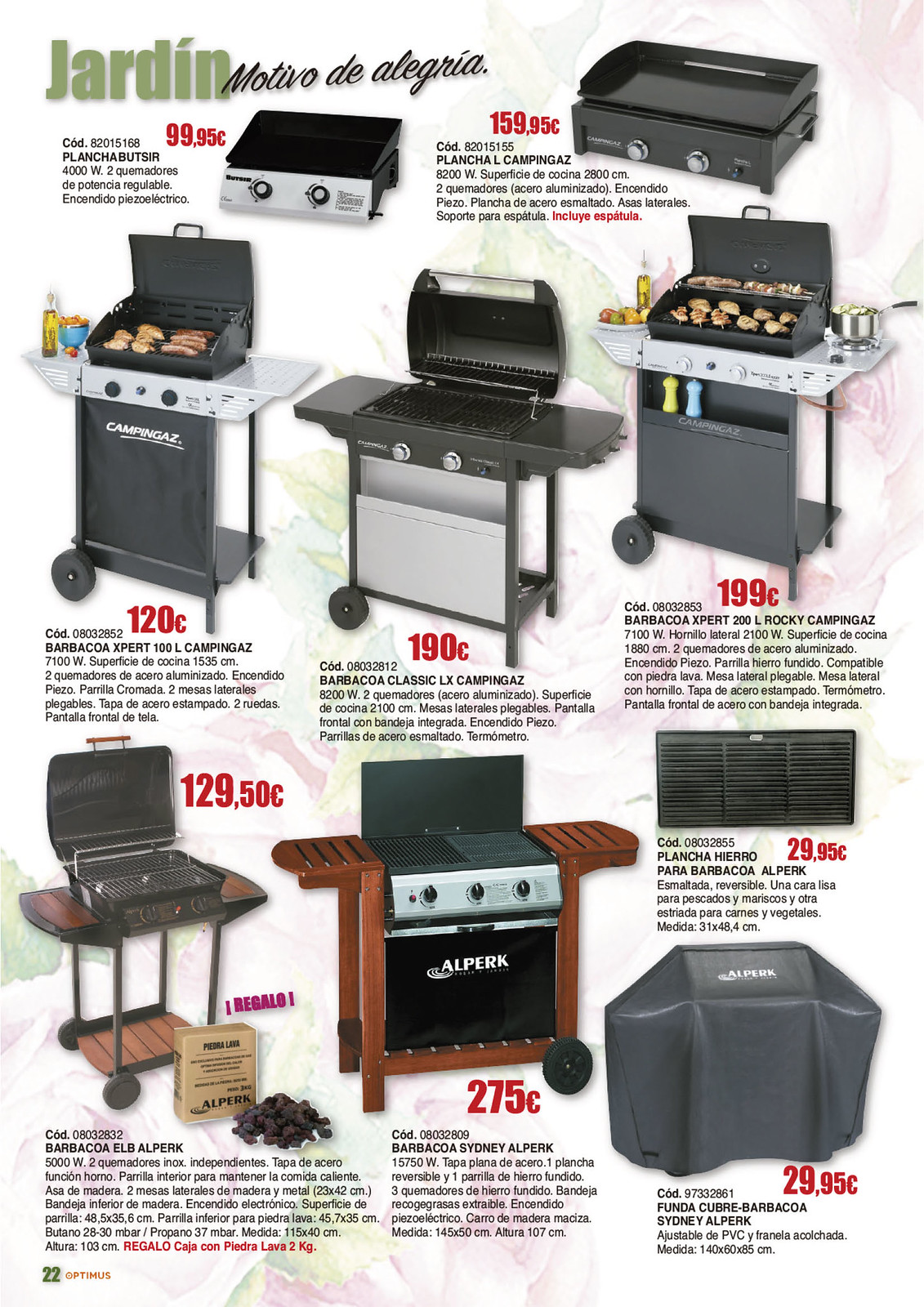The image is a highly detailed advertisement for a variety of barbeque grills and accessories presented in a catalog format, written in Spanish. The top left corner of the page features the title "Jardin Motivo de Alegría," indicating a joyful garden theme. The page number "22" is marked in green, and the word "Optimus" is prominently displayed in red.

The advertisement showcases a range of barbeque grills, with prices listed in Euros. The top two products are small indoor grills, including one labeled "Plancha" priced at 99.95 euros and another "Plancha Campingas" at 159.95 euros. These small grills are ideal for indoor use.

In the middle section, three large outdoor grills are displayed. The first is a full-standing barbeque grill with a silver base and an open black lid, labeled "Barbacoa Expert 100," priced at 120 euros. This grill features side plates holding items like a bottle of olive oil. The second is an all-black standing grill, labeled "Barbacoa Classic," priced at 190 euros, noted for its simplicity and absence of food display. The third is another large standing grill, featuring a mix of silver and black, labeled "Barbacoa Expert 200," and priced at 199 euros. This grill has food on display, including meat and vegetables, and additional items like a pot and salt and pepper shakers.

Towards the bottom, the two left-most products are identified as old-style outdoor grills. One features a wood finish on the side plates and bottom, labeled "Barbacoa EOB," but it does not have a listed price. The other is a black grill with a silver plate and knobs, framed with wooden elements and a black apron in front. It's labeled "Barbacoa Sydney Alperc," and priced at 275 euros.

On the right side of the advertisement, there is a grill part labeled "Plancha Herrero," priced at 29.95 euros, and below it is a black grill cover labeled "Funda Cubre Barbacoa," also priced at 29.95 euros. The various barbeque brands featured include Alperc and Campingaz. 

This catalogue page combines a diverse selection of grilling solutions and accessories tailored for both indoor and outdoor barbeque enthusiasts.